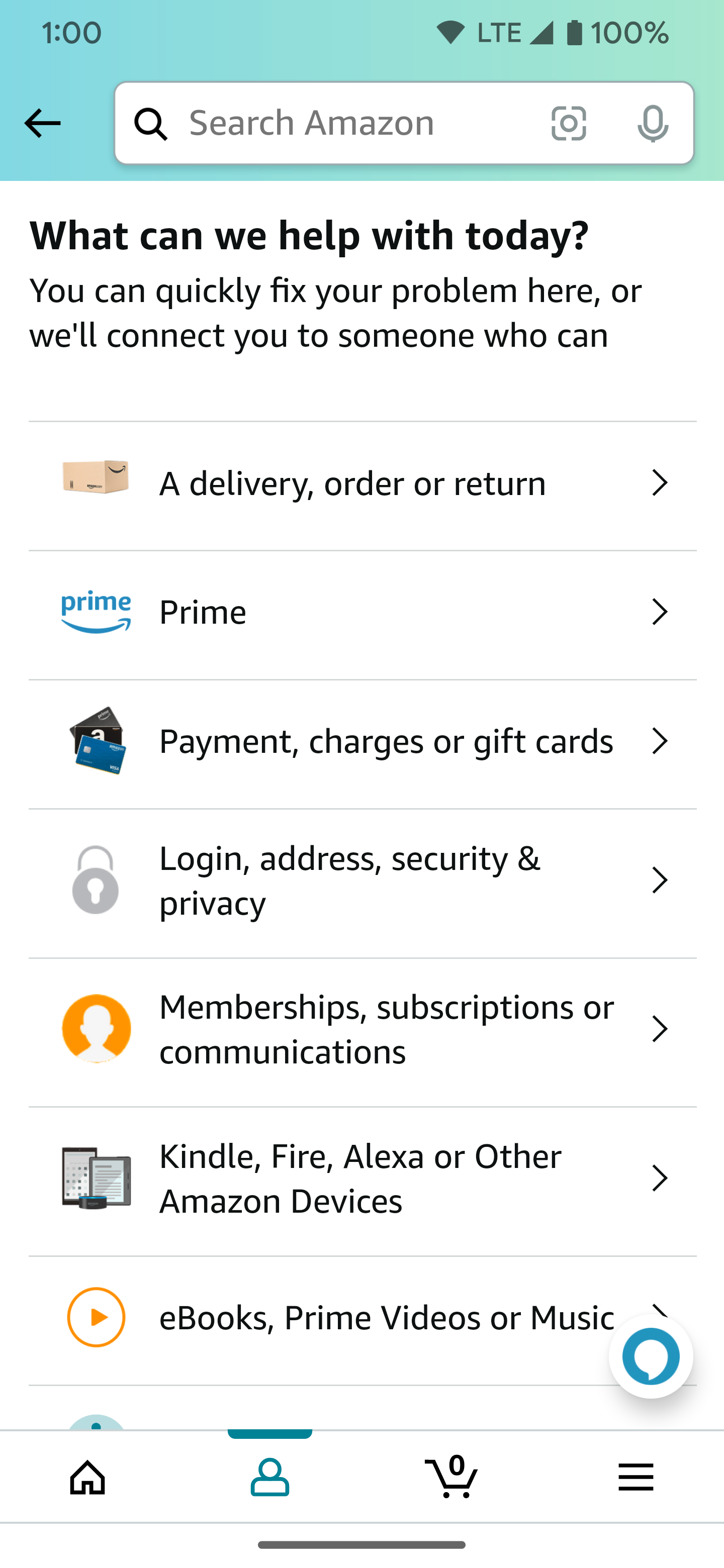This image is a detailed screenshot from the Amazon mobile application, captured in portrait orientation. The screenshot is from a device with the status bar showing at the top, featuring a light blue background similar to the color of the Amazon logo. The status bar includes the time at 1:00, a fully connected Wi-Fi icon, LTE letters with a full network connection meter, and a fully charged battery at 100%.

Below the status bar, on the left, is a left-pointing arrow situated next to a rectangular white search bar labeled "search Amazon." Immediately underneath, the page has a white background with a black header that reads: "What can we help you with today." Following this, it says, "We can quickly fix your problem here or we'll connect you to someone who can."

Next, the page displays a series of selectable options, each within its own section divided by thin gray lines at the top and bottom. Each option contains an icon on the left, a descriptive label to the right, and a right-facing caret on the far right indicating a dropdown menu. The options listed include:
1. Delivery or Order Return
2. Prime
3. Payment, Charges, or Gift Cards
4. Login, Address, Security, and Privacy
5. Membership, Subscriptions, or Communications
6. Kindle, Fire, Alexa, or Other Amazon Devices
7. eBooks, Prime Videos, or Music

At the very bottom of the screenshot, there is a white border containing icons for navigating the app. These icons include Home, Profile, Shopping Cart, and a Hamburger Menu to access additional features.